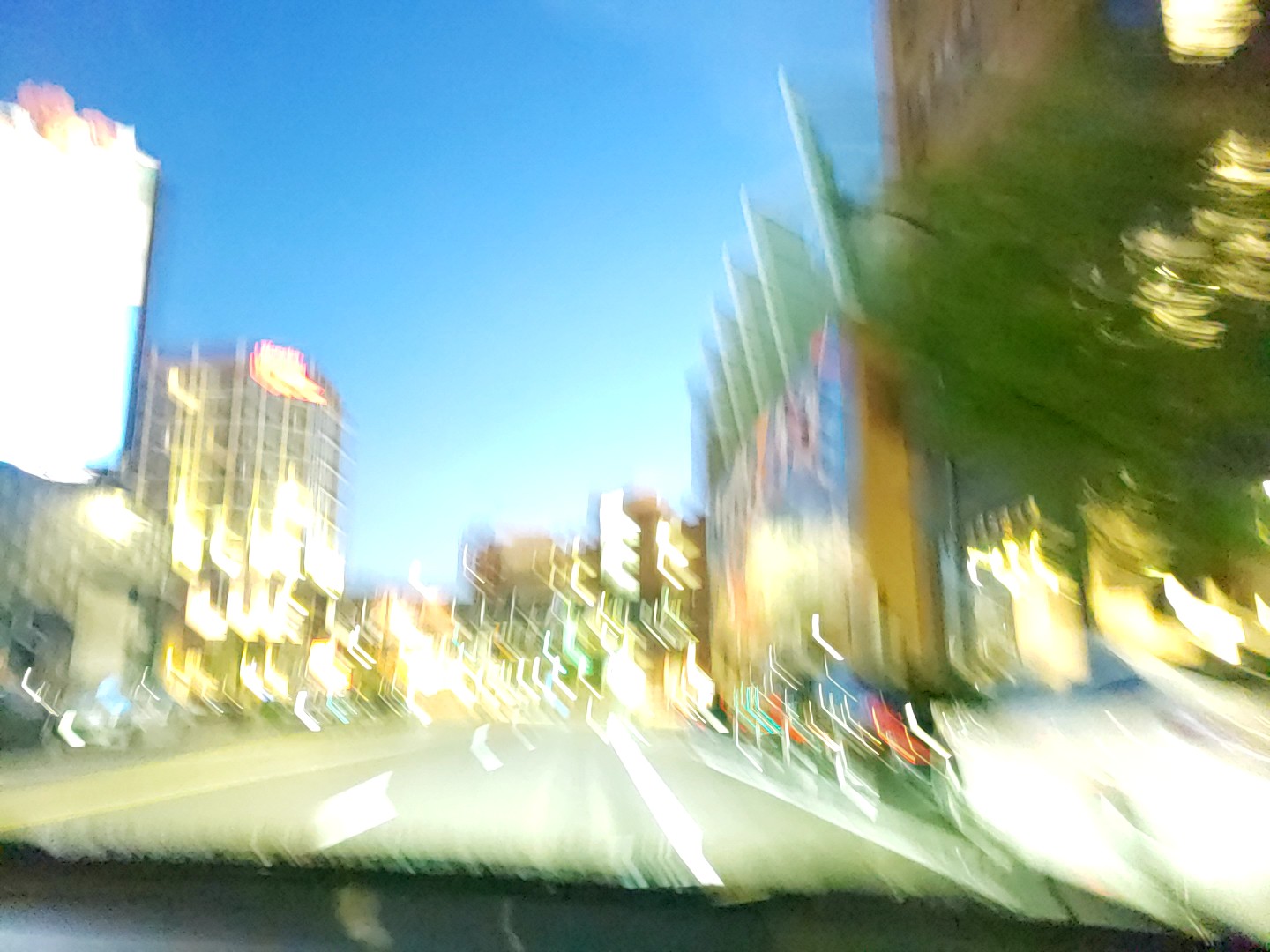This intriguing image captures the perspective of a passenger seated in the front seat of a car, traversing through a cityscape. The photo, taken from inside the vehicle, displays a blurry view as if the camera was in motion when the picture was snapped. The car is situated in the rightmost lane, with a row of parked cars lining the street to the right. Also featured on the right side of the image are a small tree and a series of imposing high-rise buildings. The scene suggests it is either dusk or after nightfall, indicated by the illuminated yellow fluorescent lights emanating from the buildings. The sky, albeit difficult to discern due to the blurry and oddly colored nature of the photo, appears to be a dark shade of blue. Notably, there are no vehicles visible directly ahead on the road, adding a sense of quiet anticipation to the urban journey.